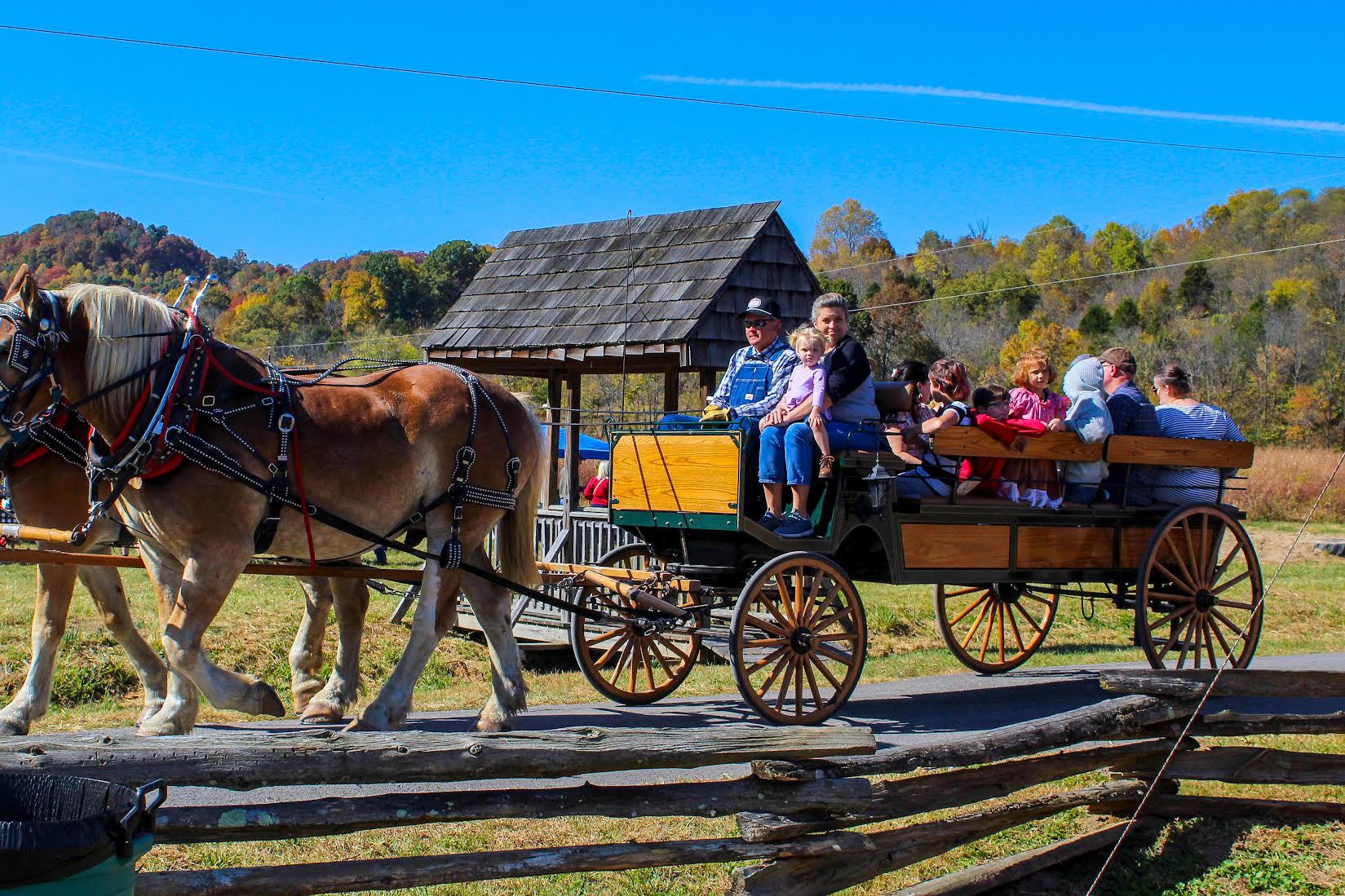This photograph captures an outdoor scene centered around a horse-drawn wagon. The wagon, constructed with a green metal frame and light wood paneling, features classic wooden spoked wheels. It is being pulled by two large Clydesdale-type horses, predominantly brown with lighter legs, and the closer horse has a mane of white hair. Sitting at the front of the wagon, a man in blue overalls and a hat holds the reins, while a woman next to him cradles a small child on her lap. The back of the wagon is filled with about half a dozen people, mostly children, accompanied by a few adults, evoking the atmosphere of a family outing akin to a hayride.

The surroundings enhance the rustic charm of the scene, with a small wooden fenced building visible behind the wagon, and a covered bridge running perpendicular to their paved path. This path is bordered by grass and a simple wooden fence. The backdrop features a rolling hill, a series of trees, and a vibrant blue sky, suggesting a peaceful countryside or possibly a cider mill setting.